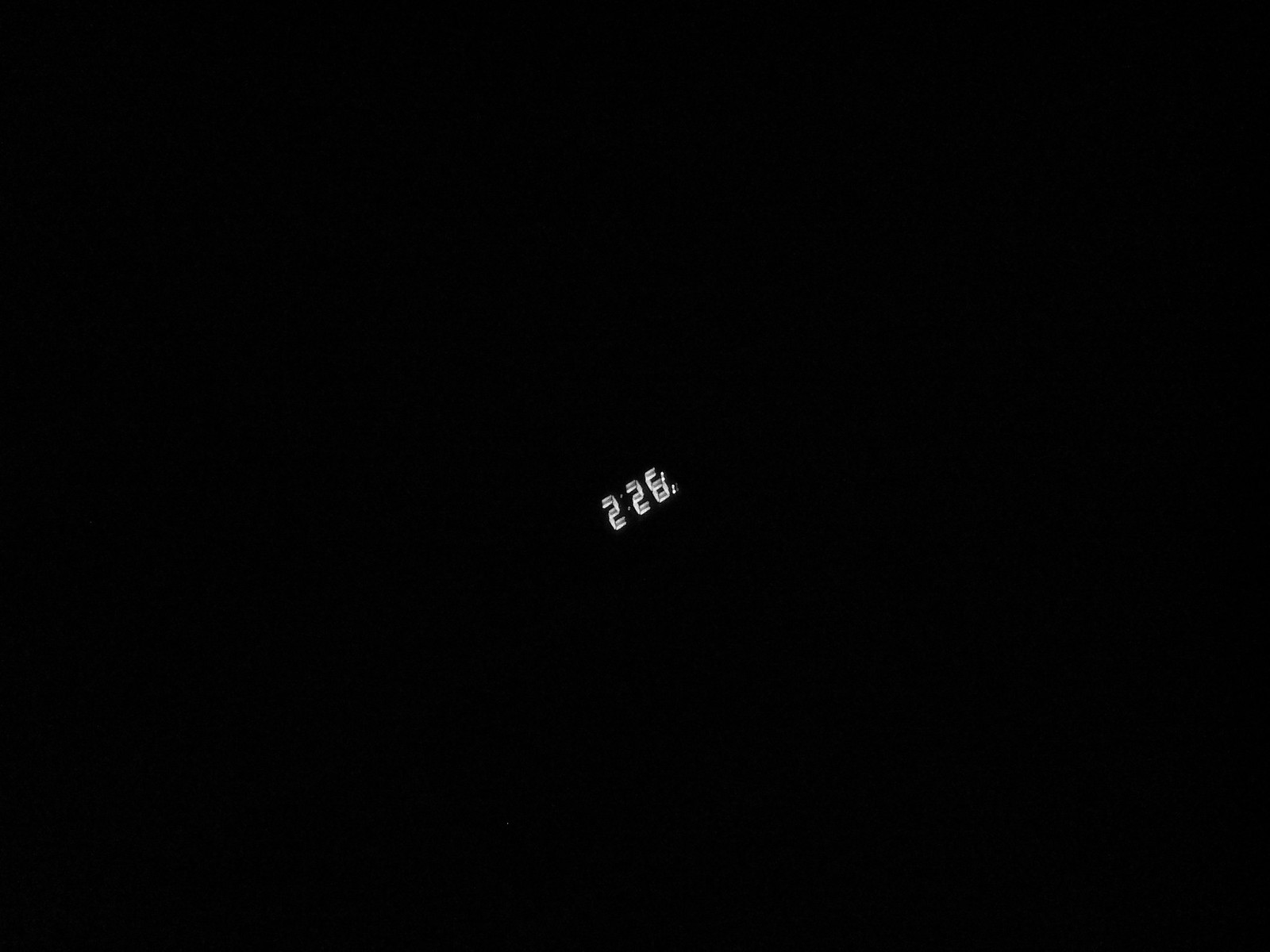A black image is centered with a slightly blurred digital clock display in white, showing the time "2:26". The numbers are positioned at an upward angle from left to right and appear as a faint double image, creating a subtle ghosting effect. To the right of the number "6," there are two barely visible dots. The entire digital display is small, occupying a minimal portion of the image, making the tiny characters stand out amidst the dark background. If the numbers were any smaller, they would become difficult to read.